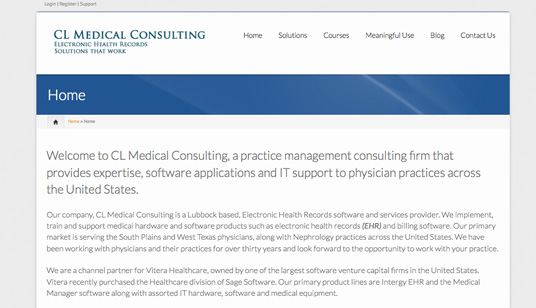Screenshot of the CL Medical Consulting website's homepage. At the top, the title reads "CL Medical Consulting, Electronic Health Records, Solutions at Work." To the right, the navigation menu includes options such as Home, Solutions, Courses, Meaningful Use, Blog, and Contact Us.

A dark blue banner features prominently, with the word "Home" in white lettering. Below this banner, a detailed introduction welcomes visitors to CL Medical Consulting, describing the firm as a Lubbock-based practice management consulting company providing expertise, software applications, and IT support to physician practices across the United States.

The text highlights the company's offerings, which include the implementation, training, and support of medical hardware and software products like electronic health records (EHR) and billing software. The primary market areas served are the South Plains and West Texas physicians, as well as nephrology practices nationwide.

With over 30 years of experience working with physicians and their practices, CL Medical Consulting expresses enthusiasm for the opportunity to collaborate with new clients. The company is a channel partner for Viterra Healthcare, which recently acquired the healthcare division of Sage Software. Their main product lines include Intergy EHR and the Medical Manager software, along with various IT hardware, software, and medical equipment.